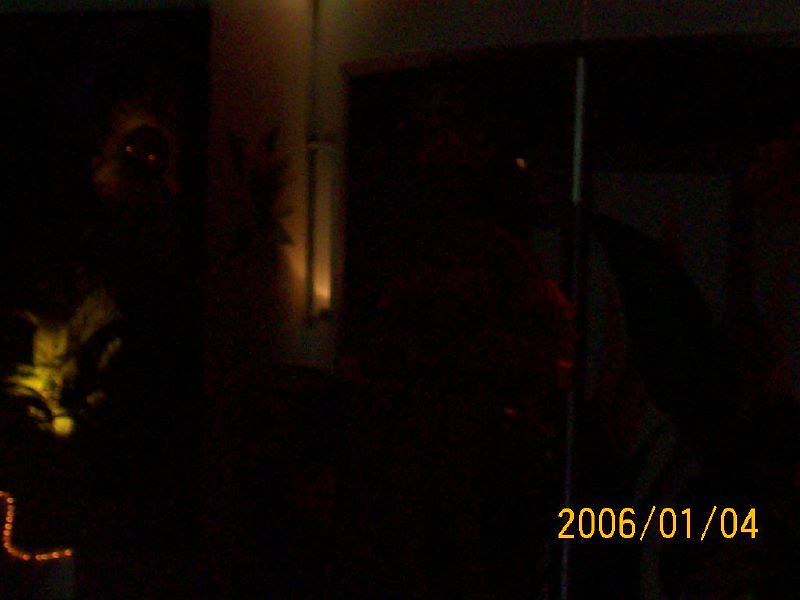In this predominantly dark and grainy image, captured at night and timestamped January 4, 2006, a few faint light sources subtly illuminate parts of the scene. Near the lower left corner, a shrub or fern appears bathed in a subdued light, with an orange, squiggly illuminated line extending from the left edge and then curving right before ending. A distinct light shines up on the side of a building, casting a yellowish hue on its surface. This building light also partially illuminates what looks like a brownish, animal-like mask or statue with a bronzed nose and flared eyes.

Just left of the center, two red dots—perhaps eyes—emerge from the darkness, seemingly belonging to a person or a figure wearing a mask, their gray or white hair faintly visible. Some light reflections suggest possible white blinds on a back wall, but the details are ambiguous due to the darkness. The right side of the image remains largely featureless, enveloped in inky blackness.